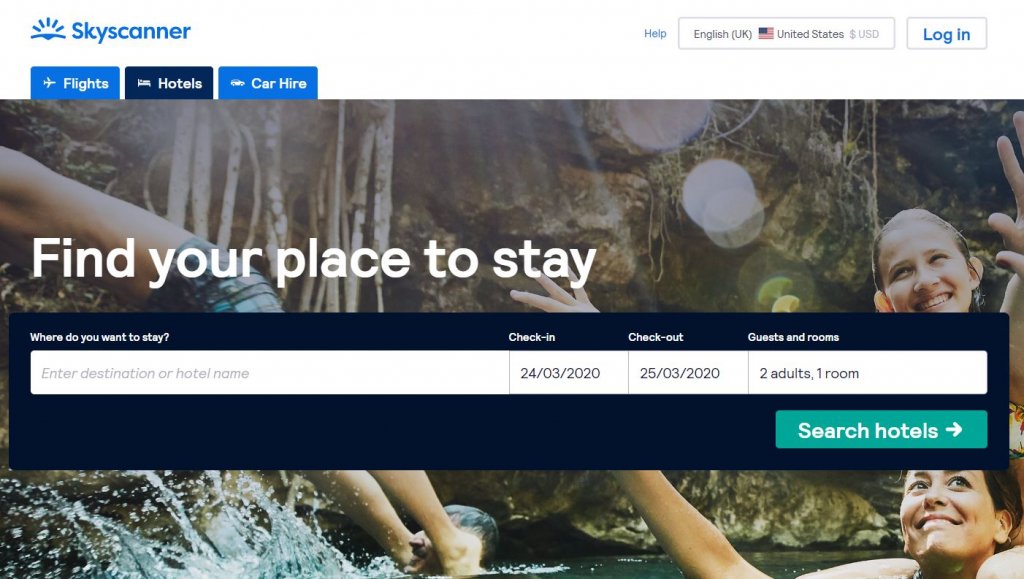This screenshot captures the homepage of the Skyscanner website.

In the top left corner, the logo comprises a blue horizon and sun, followed by the name "Skyscanner." The top right corner features navigation options including a blue 'Help' link, a language selector displaying "English (UK)," an American flag icon labeled "United States," and the currency indicator showing "USD" for US dollars.

To the far right is a link to 'Log In.' The upper left offers three main options: 'Flights' (marked by a small airplane icon), 'Hotels' (marked by a small bed icon), and 'Car Hire' (marked by a small car icon). The active page is ‘Hotels,’ signified by a navy blue background on that button, contrasting with the lighter blue on the other buttons.

Dominating the page, white text reads "Find your place to stay" over an image of a family playing in a lake or pond. Below this, a navy blue box contains an extensive search bar. The bar prompts users with "Where do you want to stay?" while placeholders within it suggest entering a "destination or hotel name." Adjacent fields allow users to specify "Check-in" and "Check-out" dates, "Guests" and "Rooms," with a teal button for submitting the search.